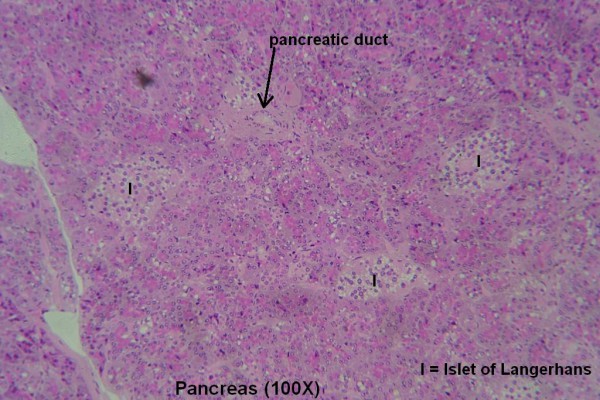This highly magnified image, approximately 100 times zoomed, features a zoomed-in view of a pancreas, as indicated by the label "pancreas (100x)" in black font at the bottom. The background is a textured purple, speckled with various shades of purple, white, pink, and even hints of brown and blue. A black downward-pointing arrow at the center top, labeled "pancreatic duct," directs attention to a lighter purple region. Scattered throughout the image are dark to light purple and white speckles, possibly representing varied tissue components. In the bottom right corner, black text reads "I = Islet of Langerhans," referring to a specific pancreatic structure. Additionally, dark black lines meander across the image, suggesting details of the inner structure. The top left corner also contains a minor brown speckle. Overall, the intricate details suggest a complex internal view of the pancreas, capturing its nuanced texture and structure.